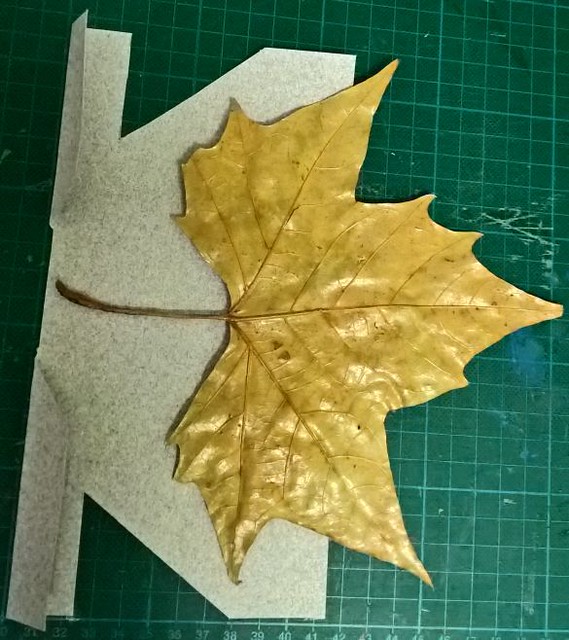The image depicts a large golden leaf, possibly a statue or crafted item, centrally positioned against a green background with a white grid pattern resembling graph paper. At the bottom, a scale with white numerals ranging from 31 to 50 is visible, suggesting a measuring tool. To the left, the leaf is resting on a gray, spotted material, resembling folded paper. The setting appears to be indoors, potentially a classroom, characterized by a combination of turquoise, white, gray, gold, and brown hues. The leaf is intricately detailed, with golden veins and a brown stem, emphasizing its artistic depiction.